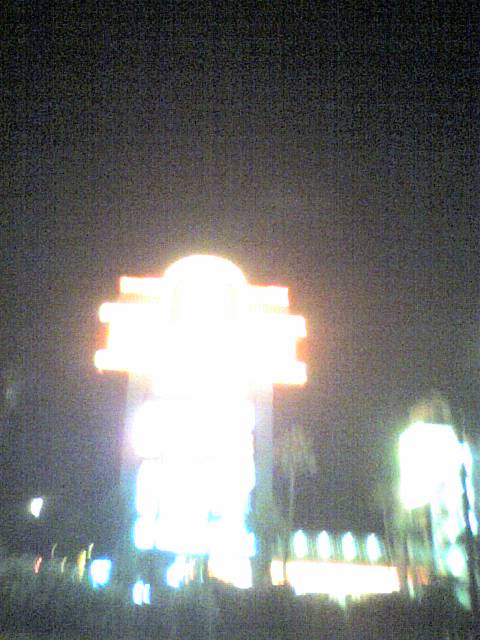The image depicts a large, blurry, and grainy digital sign, illuminated predominantly in yellow-orange at the top and blue towards the bottom, likely enhanced by neon lights. Positioned prominently in the image, this sign contrasts with a smaller, greenish neon sign located to its right. Between these signs stands a slender tree, and a well-lit building can be seen in the background. The overall scene is dark, suggesting it was captured either at dusk or during the night. Below the signs, there are some bushes adding to the scenery.